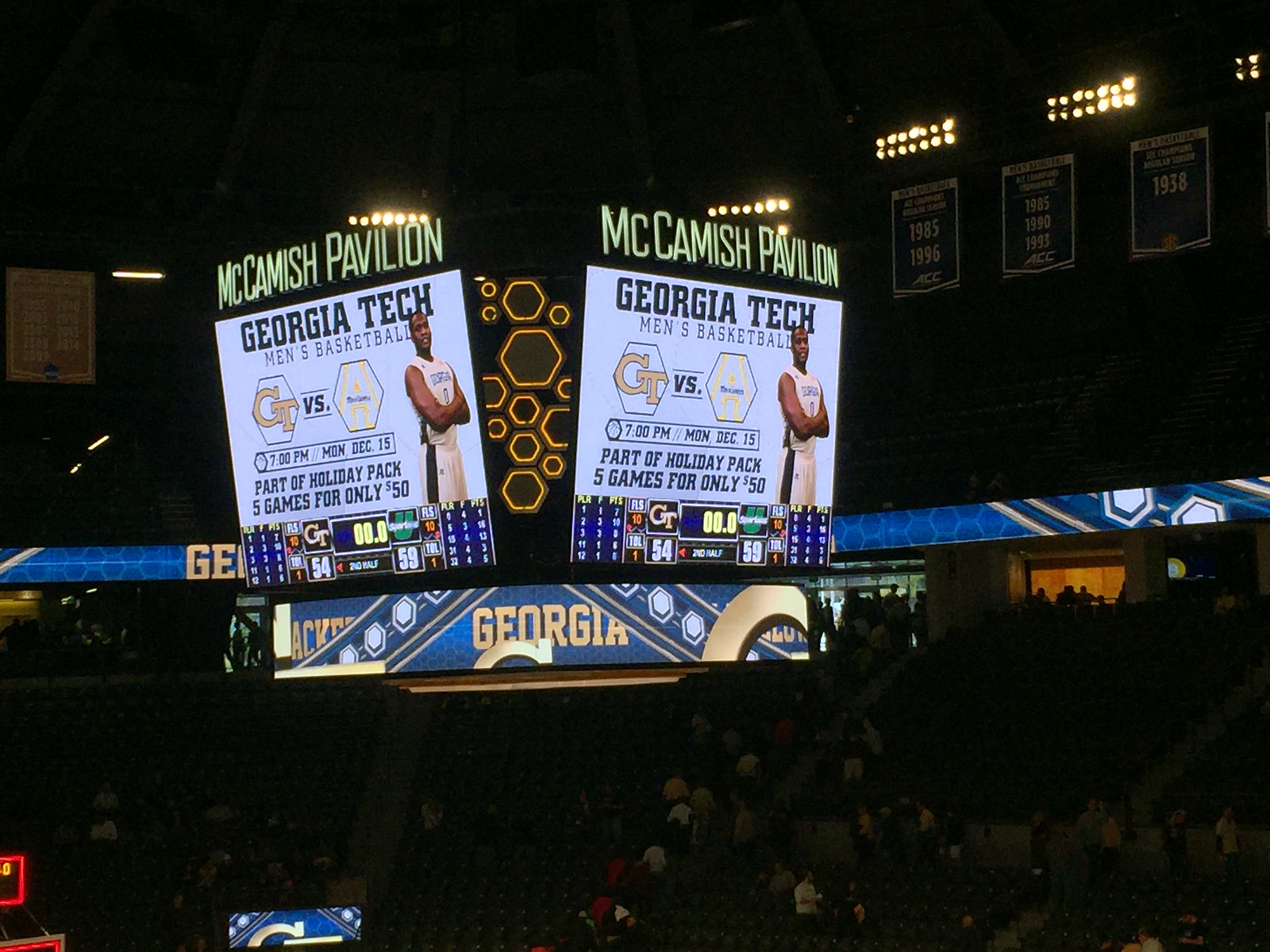The image captures the bustling aftermath of a basketball game at McCamish Pavilion. Spectators are seen dispersing towards various exits from both the lower and upper decks of the stadium. Dominating the center of the image is a large jumbotron-like scoreboard with multiple screens. The scoreboard prominently displays the text "McCamish Pavilion" above an image of a Georgia Tech basketball player, alongside the announcement "Georgia Tech Men's Basketball GT vs [unreadable opponent]." Beneath this, in fainter letters, it reads "Men's Basketball," and further down a banner indicates a promotion, "Holiday Pack - Five games for only $50."

The scoreboard also shows the game's final score with Georgia Tech scoring 54 points and their opponent 58 points. The structured arrangement of the image places the brightly lit scoreboard centrally, framed by the darker, sparsely populated seating areas of the arena. The color palette of the image is predominantly blue, black, and gold, which accentuates the illuminated elements of the stadium, including scattered lights along the top edges and a lighted strip beneath the upper deck seats. In the upper right corner, banners hang from the rafters, contributing to the arena's atmospheric depth. Overall, the setting details a concluded basketball game with departing fans amidst a well-lit and organized stadium environment.